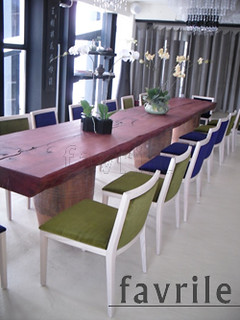In this professional advertisement image, a rustic-yet-modern office or meeting room is depicted with a prominent long, rectangular table made of reddish-brown wood featuring visible wood grains, suggesting a cherry-like finish. The table, supported by three chunky, cylindrical wooden pillars, is surrounded by a symmetrical arrangement of chairs: two green fabric chairs at both ends, flanked by three blue fabric chairs on each side, all with white frames. The green and blue fabric seats and backs stand out against the stark white chair frames, providing a vibrant yet cohesive look. 

In the middle of the table are two lush green plants, adding a touch of nature to the setting. The table and chairs are set on a light gray, white marble-like tiled floor which enhances the overall elegance of the room. To the back left of the image, large floor-to-ceiling windows let in natural light, hinting at a cityscape outside, while further back, a dark gray accordion-style curtain hangs, providing a modern touch. 

In the bottom right-hand corner of the image, the word "FAVRILE" is printed in gray, right-justified, underscored by a thin line matching the font color, possibly indicating the brand or designer of the furniture set. Hanging from the ceiling are subtle, indistinct fixtures that add a finishing touch to this stylish and minimalist interior space.